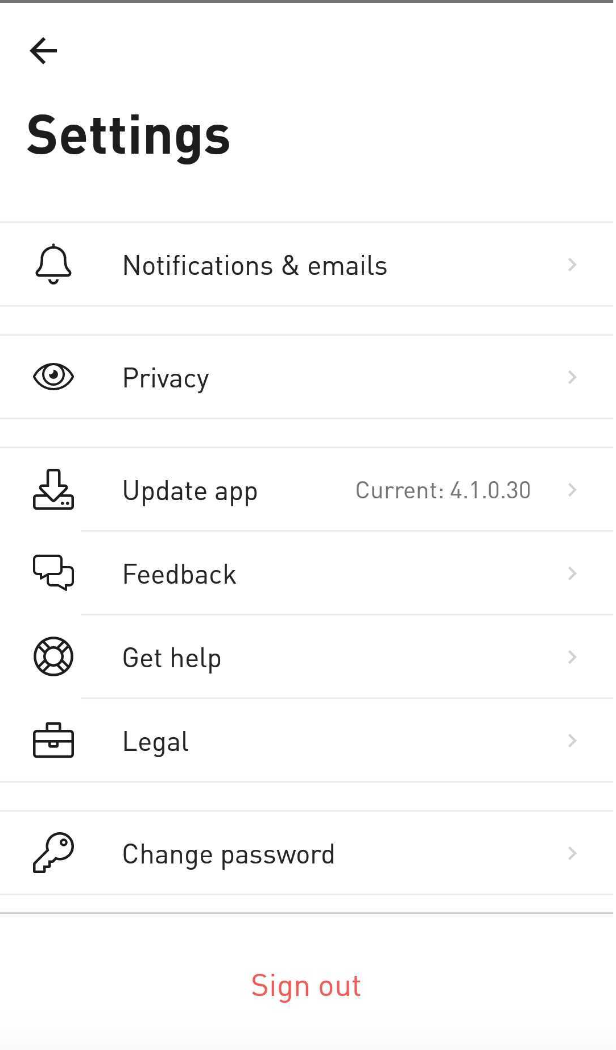The image displays the settings interface of a computer program. At the top, there is a black back arrow above the bold heading "Settings," which is in black text against a white background. The first option listed is "Notifications and Emails," indicated by a bell icon. This section allows users to configure their preferences regarding notifications and emails. Below that is the "Privacy" setting, symbolized by an eyeball icon, where users can adjust their privacy configurations.

Further down, there is an "Update App" option with a download icon, alongside information about the current app release version. The menu also includes a "Feedback" button for user suggestions, a "Get Help" button for assistance, and a "Legal" section for legal information. Near the bottom, a key icon represents the password change option, allowing users to modify their password. Finally, at the very bottom of the page, red text reads "Sign Out," providing an option for users to log out of the application.